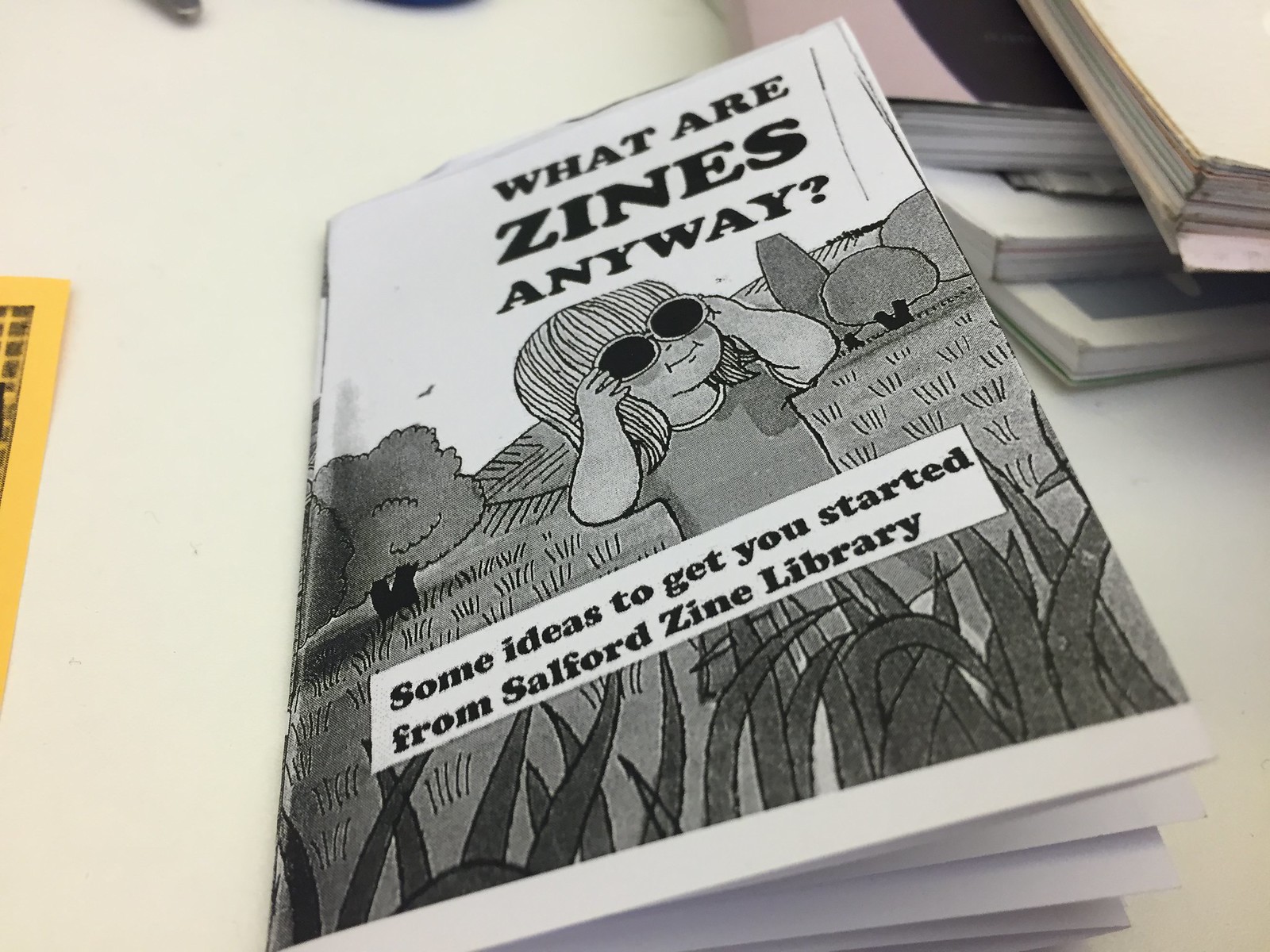The image shows a small, black and white booklet titled "WHAT ARE ZINES ANYWAY?" in bold, uppercase lettering. The cover features a cartoon illustration of a young girl with long hair, smiling as she puts on a pair of sunglasses. She is standing in a grassy field with tall blades of grass, and there are short bushy trees and a white sky in the background. Below the illustration, in a white rectangle, it reads "Some ideas to get you started from Salford Zine Library." The booklet is placed on a white table. To the left of the booklet is a yellow flyer, while in the upper right corner of the image, there are stacks of more books. The books in the pile appear to vary in color and condition, with some being worn and discolored.